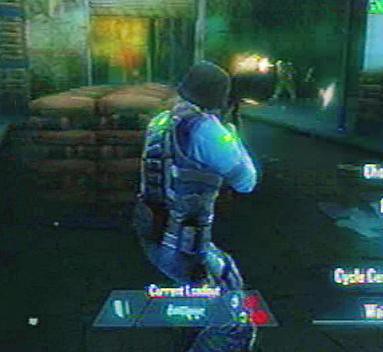This square photo is a slightly out-of-focus partial screenshot from a video game. The image features the back of a character clad in detailed armor, including a vest, various pouches, leg armor, and a round helmet. The character is positioned at the left side of the image, aiming a firearm towards a large hallway to the right. The hallway resembles a garage door opening within an industrial setting, indicated by plastic flaps hanging from a doorway to the left. In the foreground, large sacks, possibly containing feed or other goods, are stacked on a pallet. A rectangular bar spans the bottom of the screen showing partially obscured text, with only a name visible at the top. White text also appears on the right side of the screen, though it is cut off in this image.